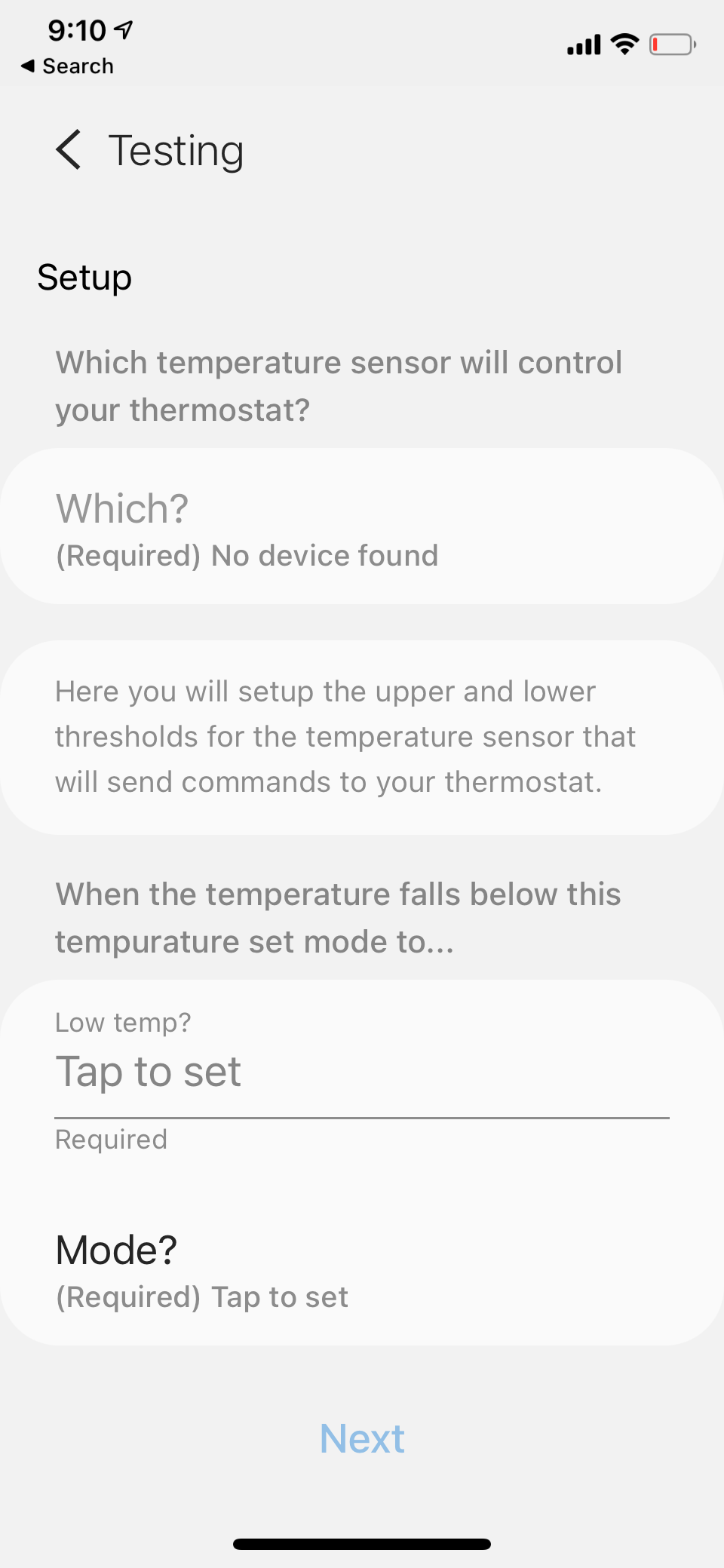The image is a screenshot of an iPhone display. In the top left corner, the time is shown as 9:10. On the top right, the network status indicates full signal strength with 4 out of 4 bars, and the Wi-Fi signal strength is also full with 3 out of 3 bars. Next to these, the battery icon is visible.

The main content of the screenshot involves setting up a temperature sensor for a thermostat. The text describes the process of selecting which temperature sensor will control your thermostat, highlighting that no device is currently found. Below this, instructions are provided for setting the upper and lower temperature thresholds that the sensor will use to send commands to the thermostat. There is a prompt indicating that setting the mode is required, with options to tap and configure accordingly.